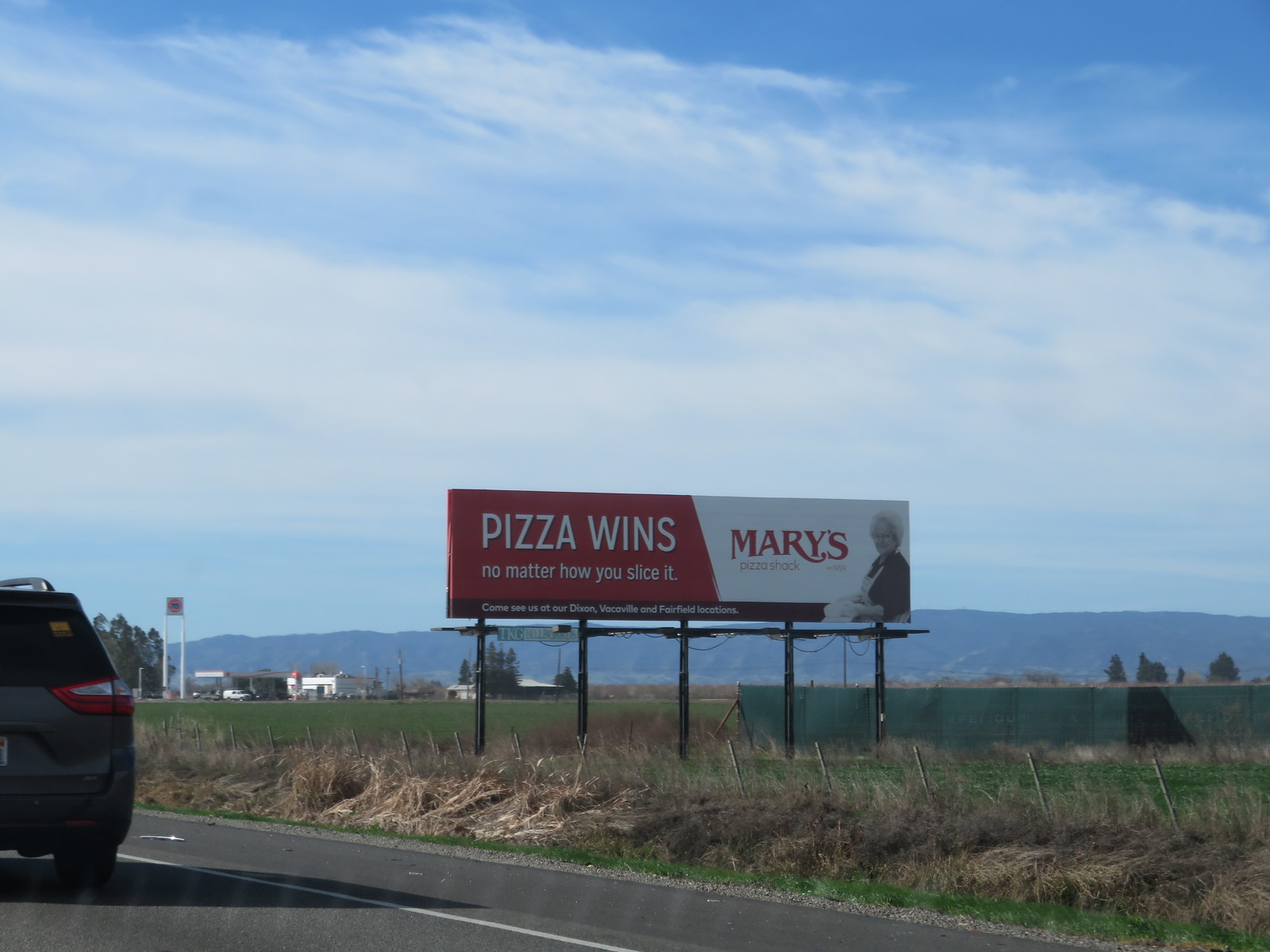The photo captures a scene of a rural highway where a person, presumably from within another vehicle, takes a picture of a large rectangular billboard supported by five black poles. The billboard prominently features a red and white color scheme. On the left side, which is red, it reads "Pizza Wins, no matter how you slice it" in white text. To the right, the billboard transitions to a white background displaying the name "Mary's Pizza Shack" in large, stylish cursive, particularly noticeable in the distinctive "R." Additionally, there is a small red text stating "Pizza Shack," and below that, an image of an elderly woman with white hair, wearing glasses and an apron, presumably making pizza. 

The lower section of the billboard has a black banner inviting people to "come see us at our Dixon..." with the rest of the text unclear. The surroundings include green and brown grass, a green metal fence at the base of the billboard, and a partially visible gray minivan with a luggage rack and an orangish-yellow sticker on its rear windshield driving by on the highway. The highway shows gray asphalt with white lane markings. In the distance, you can make out loose white clouds against a blue sky, a dark mountain range, and various indistinct buildings. There's also a gas station identified by a "76" sign.